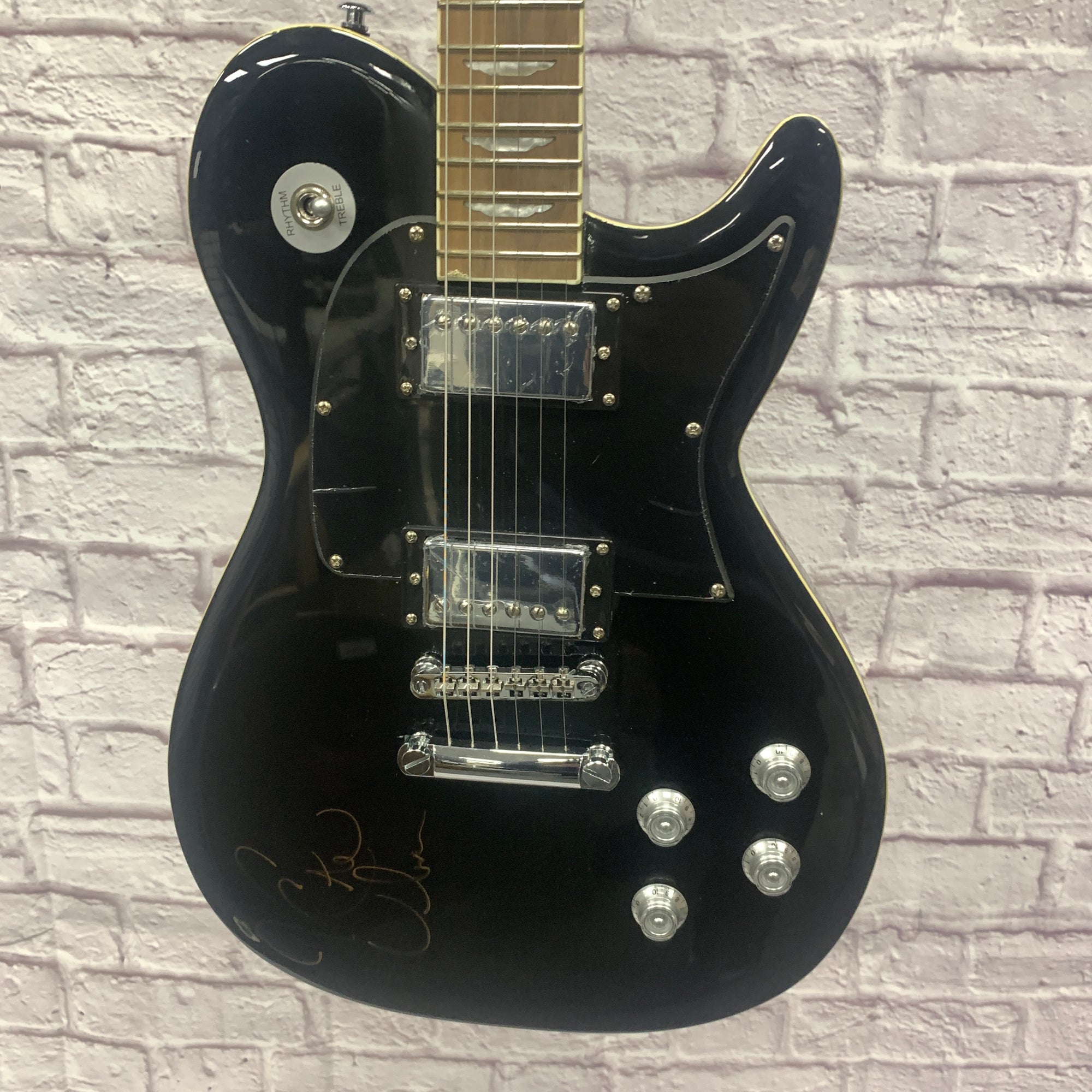This full-color photograph, taken indoors and presented in a vertically rectangular format without a border, showcases a striking black electric guitar prominently set against a painted white brick wall composed of small, square bricks. The guitar, a Fender Urban single cut model, commands attention with its sleek black body that features a distinct curvy design, rounded at the bottom and flaring into pointed ends on either side. The pickguard and signature pickups are a gleaming silver, matching the silver base where the strings are anchored. A notable feature is the silver switch adorned with a round silver plate on the upper left side of the guitar's body. The lower right corner is equipped with four shiny silver knob adjustment dials. The neck of the guitar, crafted from light brown wood and embellished with pearl inlays, extends upwards though not fully visible in the frame. Adding a personalized touch, a gold signature, likely that of Keith Urban, graces the lower left side of the guitar, making it a beautiful and unique instrument.